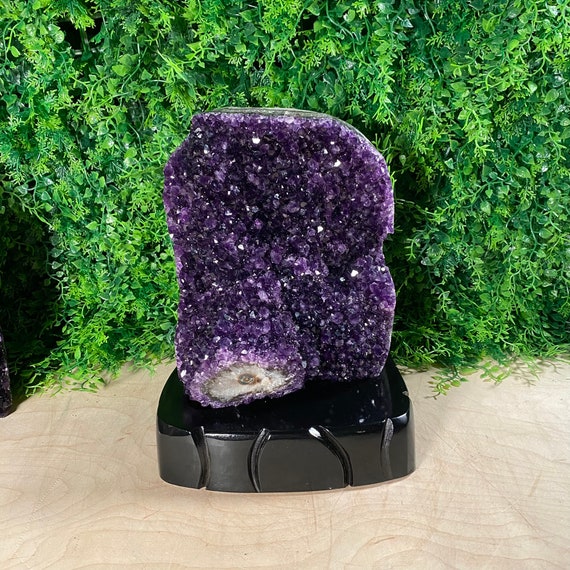This detailed photograph showcases a large amethyst geode, predominantly dark purple with intricate crystalline structures. The geode, approximately a foot tall and 11 inches wide, rests on a black pedestal that is suggested to be made of a shiny, possibly plastic material. At the base of the geode, there is an exposed section revealing white crystal formations, adding a contrasting element to the predominantly purple crystalline surface. The pedestal features decorative indentations on the sides, and the entire setup seems to be situated outdoors. The background is adorned with green foliage that appears somewhat artificial, though it is likely real. The base is placed on a tan, stone-like surface, which might be a swirled wood-patterned table. The vivid backdrop and the carefully positioned amethyst geode create a visually striking and aesthetically pleasing composition.